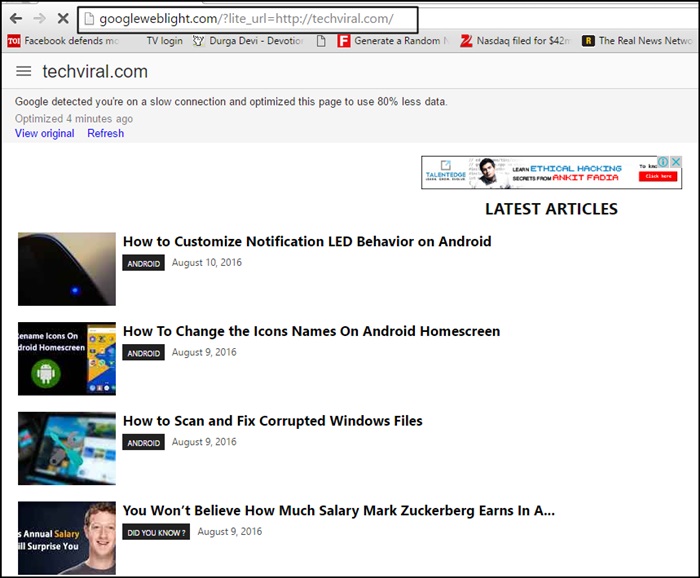A screenshot of a web browser displaying the website "techrival.com" has been optimized through Google Web Light due to a slow internet connection. The URL bar shows "googleweblight.com/?light_url=http://techrival.com/" within a dark gray highlighted section. A message below the URL indicates that Google detected a slow connection and optimized the page to use 80% less data, with the optimization occurring four minutes ago. There are two links in blue text below this message: "Original" and "Refresh".

On the right side of the screen, there is a small advertisement for a course or book on ethical hacking by Ankit Padia, though the name is slightly obscured. The main content area features the "Latest Articles" section, showcasing four article thumbnails on the left with corresponding headlines to the right:

1. "How to Customize Notification LED Behavior on Android"
2. "How to Change the Icon Names on Android Home Screen"
3. "How to Scan and Fix Corrupted Windows Files"
4. "You Won't Believe How Much Salary Mark Zuckerberg Earns…"

For each article, there are buttons labeled "Android" except for the Zuckerberg article, which has a "Did You Know?" button. The publishing dates for the articles are listed as August 10th, 2016, and August 9th, 2016, respectively.